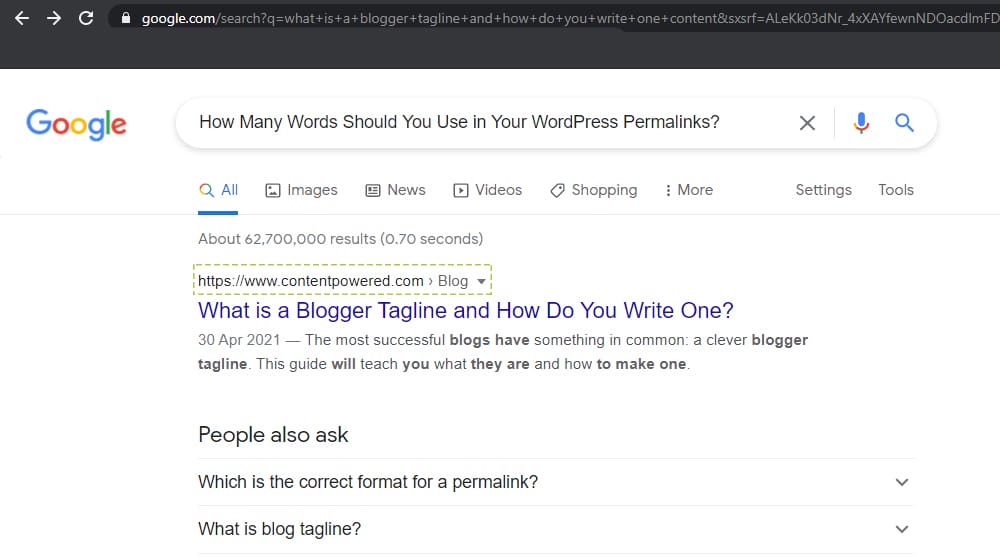The image depicts a Google search results page. At the top, a black bar displays the URL "google.com" followed by additional text. To the left of the URL, there is a padlock icon representing a secure connection, and next to it, a circular arrow icon, typically used for refreshing the page. Navigation arrows for going back and forth in the browsing history are visible on the far left.

The search query entered is "how many words should you use in your WordPress permalinks?" The query appears in blue with an underline, indicating a hyperlink. Below the search bar, various results are displayed. One highlighted result is titled "What is a blogger tagline and how do you write one?" dated April 30, 2021. The description beneath this result states, "The most successful blogs have something in common, a clever blogger tagline. This guide will teach you what they are and how to make one."

Additionally, a "People also ask" section is present, featuring expandable questions with down arrows. Two questions listed are "Which is the correct format for a permalink?" and "What is a blog tagline?" Clicking the down arrows next to these questions would reveal more information.